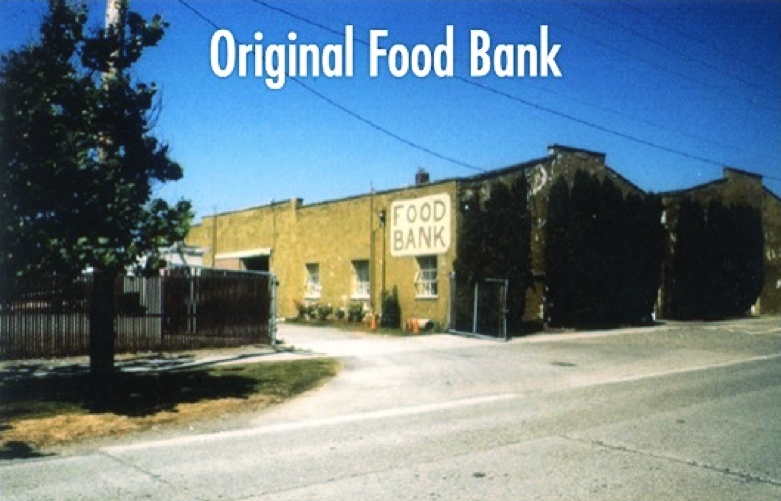This grainy, 40-year-old photograph, titled "Original Food Bank" in white letters at the top, captures a rundown industrial building against a bright blue sky. The building, likely made of beige brick, bears a large white sign with dark reddish-brown letters spelling "Food Bank" across an entire story height-wise, situated above a window. In total, there are three visible white-framed windows on the front of the building, partially cast in shadow.

The right side of the building appears severely damaged, possibly from a fire, with significant burn marks evident. To the left of the building, a prominent tree and a chain-link fence with brown and white vertical panels are noticeable, while the bottom right of the image shows the brick wall. The image is framed with electrical cords stretching across the sky and a deserted streetscape featuring a modest sidewalk and a grassy patch with potted plants beneath the windows. The scene is devoid of people or cars, suggesting an abandoned, quiet moment from a sunny day in the past.